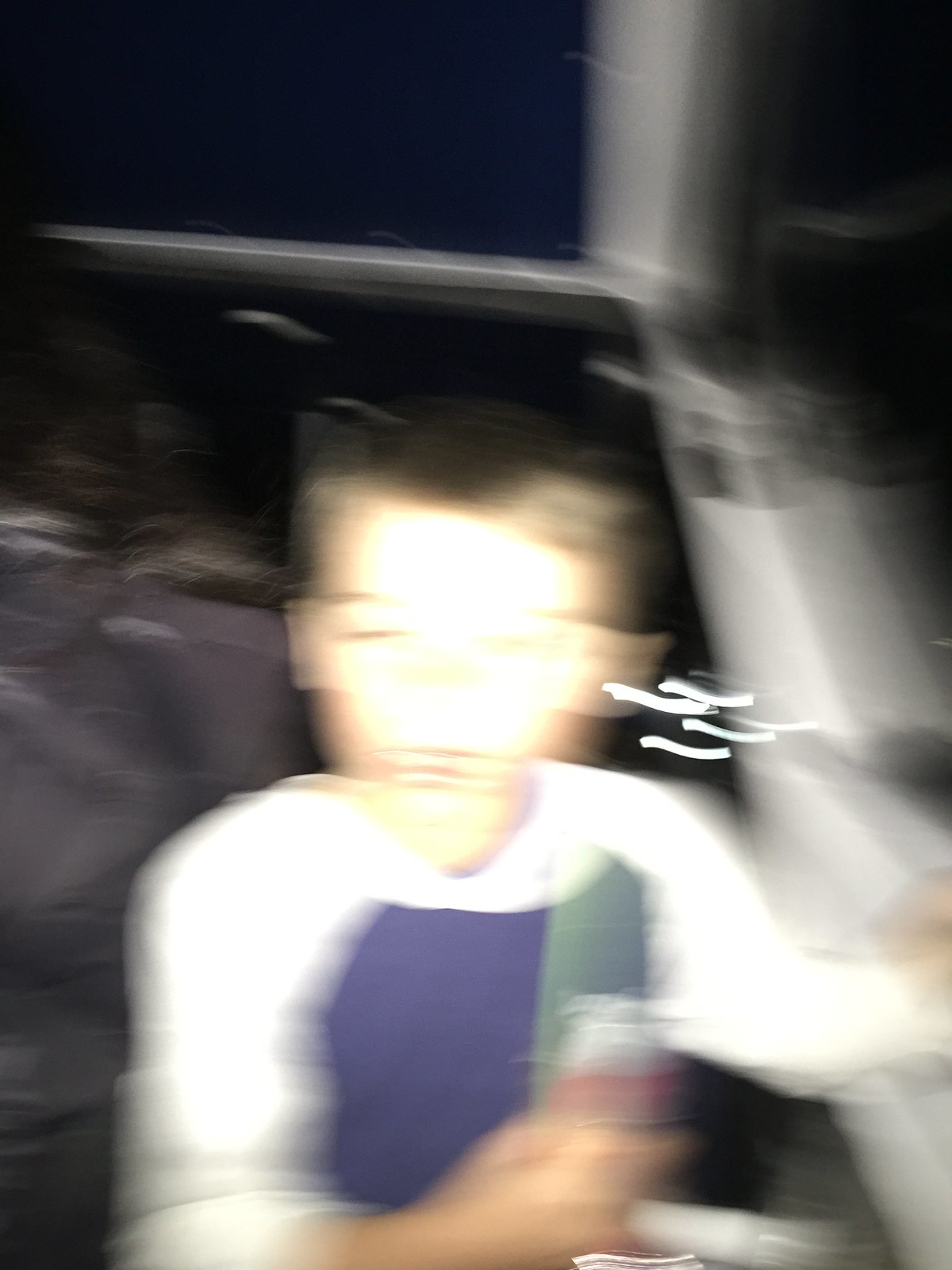This is a very blurry and grainy photo of what appears to be a young Caucasian boy, roughly seven or eight years old, with short dark hair, facing the camera. He is dressed in a long-sleeve baseball tee that is blue around the chest and white on the sleeves, pushed up to his elbows. He is sitting down on what might be a floor, possibly in his room, but the setting is unclear due to the blurriness; he could also be on stairs, a seat in a car, boat, or another form of transportation. The child is holding what seems to be a soda can, possibly Diet Coke, in his right hand, and his left hand appears to grasp a railing. The background reveals dark flooring possibly covered with blankets, blue walls with white trim and baseboards. The child's face is significantly blown out, making details hard to discern, with only a slit visible for his right eye and two red lines hinting at his mouth. Additionally, there are faint white lines near his face that look drawn on.